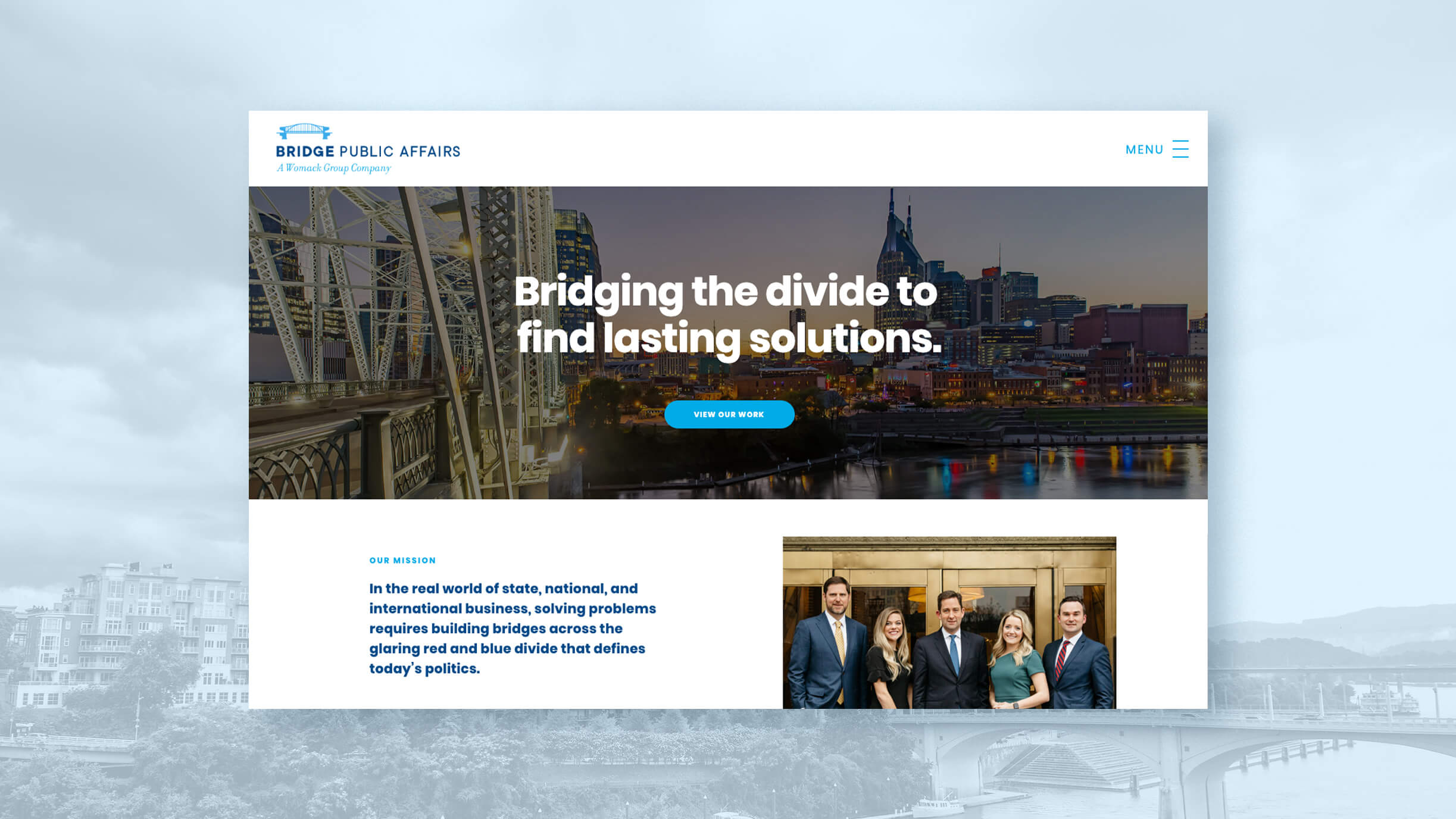The website for Bridge Public Affairs features a captivating landscape photograph as its background, showcasing buildings to the left, a bridge extending over water to the right, and a cluster of trees in the middle. The website's name, "Bridge Public Affairs," is prominently displayed in blue text. 

Below, on a white background, there's a city skyline image accompanied by the tagline, "Bridging the Divide to Find Lasting Solutions." Just beneath this tagline is a blue button labeled "View Our Work."

Further down, the section titled "Our Mission" is complemented by an image of five individuals, consisting of three men and two women, all dressed in professional business attire. The men are in suits, while the women are in what appears to be a black dress and a green dress, both showcasing long blonde hair. They stand poised in front of a building with gold-framed clear doors. The accompanying text reads, "In the real world of state, national, and international business, solving problems requires building bridges across the glaring red and blue divide that defines today's politics."